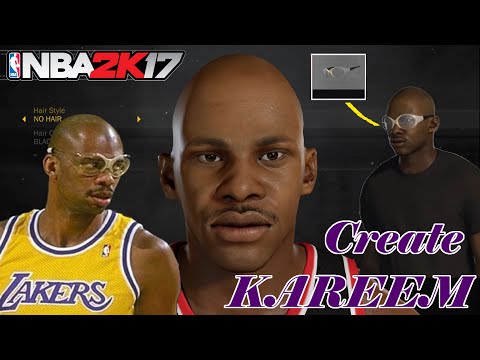A detailed in-game screenshot from NBA 2K17 showcases the "Create Kareem" feature, allowing players to customize basketball legend Kareem Abdul-Jabbar. The NBA 2K17 logo is prominently displayed in the upper left corner, confirming the game's identity. In the bottom left corner, a reference image of Kareem Abdul-Jabbar is provided to guide customization. Centrally located is the main character model in progress, while on the right, a mannequin-like figure serves as a secondary example. The user is currently selecting Kareem's iconic goggle glasses, visible in a gray pop-up box with a black bar at the bottom containing various options. Although not visible, selections are controlled via a remote, showcasing the detailed customization process for Kareem's character in the game.